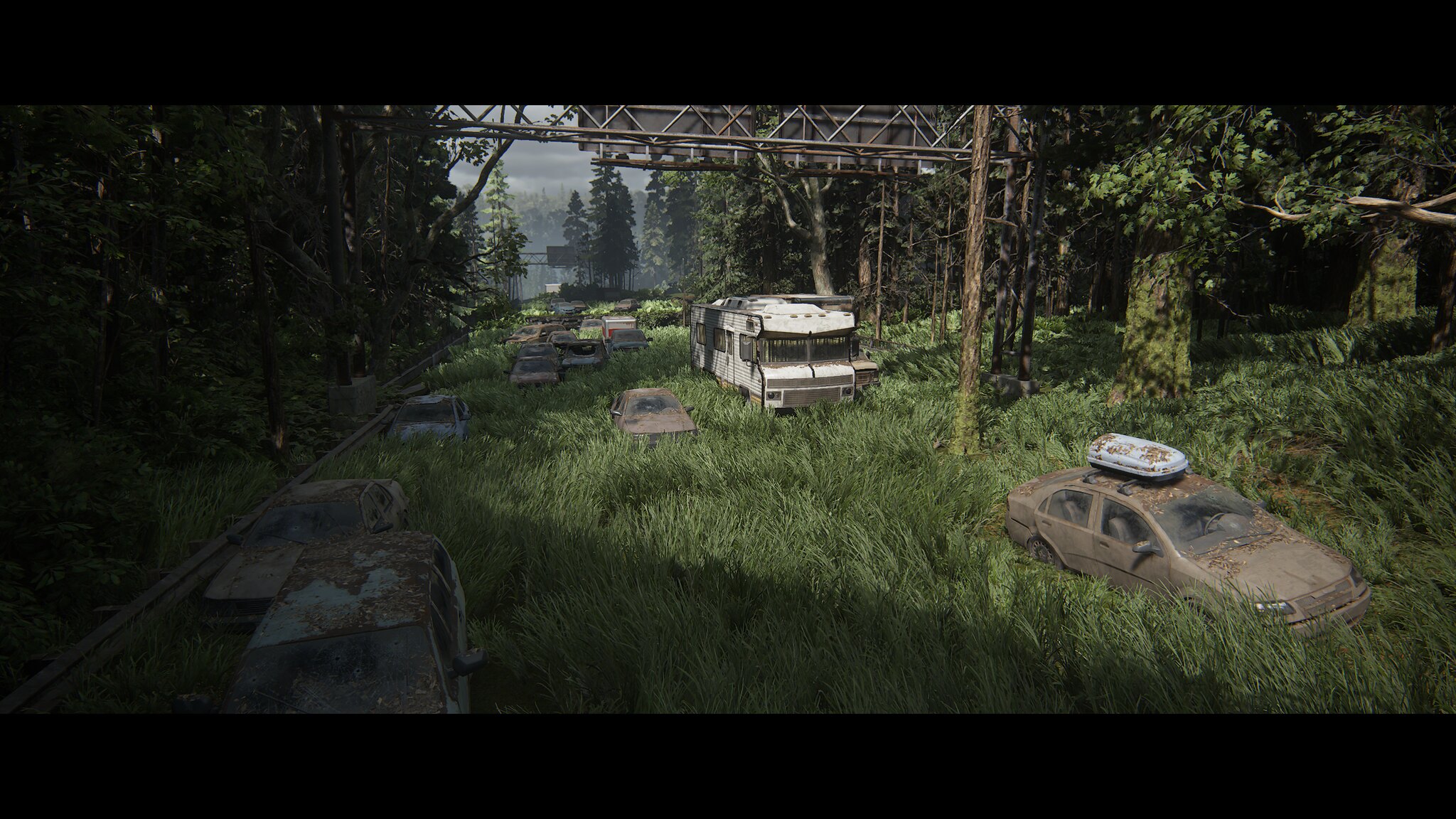The image is a screenshot from a post-apocalyptic video game, featuring a completely abandoned highway that has been overtaken by nature. Tall grass and a variety of trees, including pine, have grown over the asphalt, creating a vivid contrast of green against the dilapidated scene. The highway is littered with dirty, rusted vehicles, including a prominently displayed large white RV. This RV, along with three or four other cars, is dispersed across the now desolate freeway. The greenery encompasses the entire area with trees of different shades, casting shadows and adding to the haunting atmosphere. A highway sign looms above the RV, but from this angle, only the back of the sign is visible. The sky above is a hazy mix of blue and gray, further contributing to the scene's end-of-the-world ambiance.